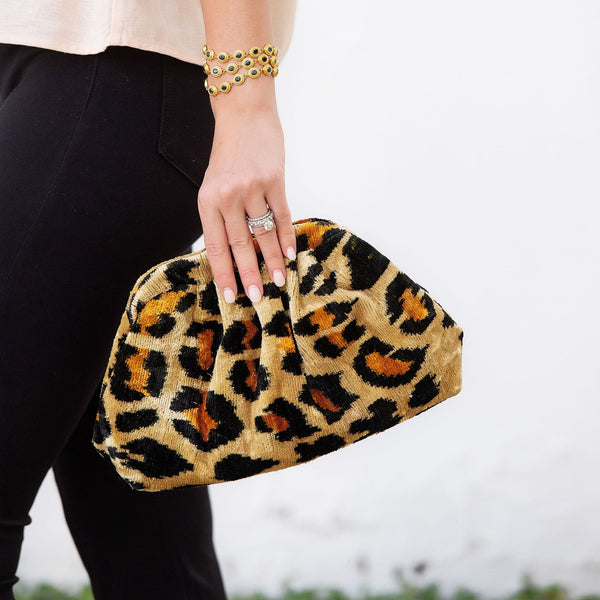This image showcases a woman walking away, cropped from the waist down. Her left leg is stepping forward, and her attire includes black jeans and a glimpse of a white blouse. Her left hand swings back, loosely holding a lightweight, medium-sized leopard print clutch handbag. The clutch, with a velvet-like texture, is the focal point of the image, suggesting it might be an advertisement. The woman's hand is adorned with a striking set of detailed accessories: an elaborate platinum-colored wedding ring, a muted white manicure, and three elegant bracelets — two jade and gold and one comprising three gold chains with jade circles. The background is a plain white, directing full attention to the handbag and accessories.